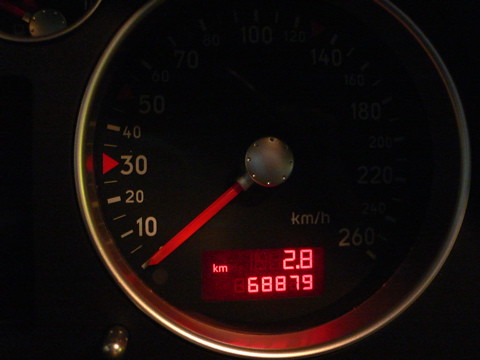This detailed photograph features a car's odometer against a dark brown or black background. The focal point of the image is the odometer dial with its striking bright red needle, which is currently positioned at the far left, indicating no movement. The dial's center point is black, and it anchors the red needle which rests peacefully at the lowest marking on the left.

Progressing from the 8 to 9 o'clock position, the gauge is marked with white or yellow numbers and lines, indicating increments of 10, 20, and 30. A distinct right-facing arrowhead points towards the number 30. At the bottom center of the circle, the abbreviation "KM" is illuminated in neon red, accompanied by two rows of numerical readings: the top row displays "2.8" and the bottom row "68,879". Above these, faint white letters spell out "KM" once more.

Additionally, at the 7 o'clock position, just outside the dial frame, a small speck of bright yellow light appears, likely a reflection adding a subtle touch to the composition. This careful arrangement of elements and the vibrant colors against the dark backdrop make the image strikingly vivid and clear.